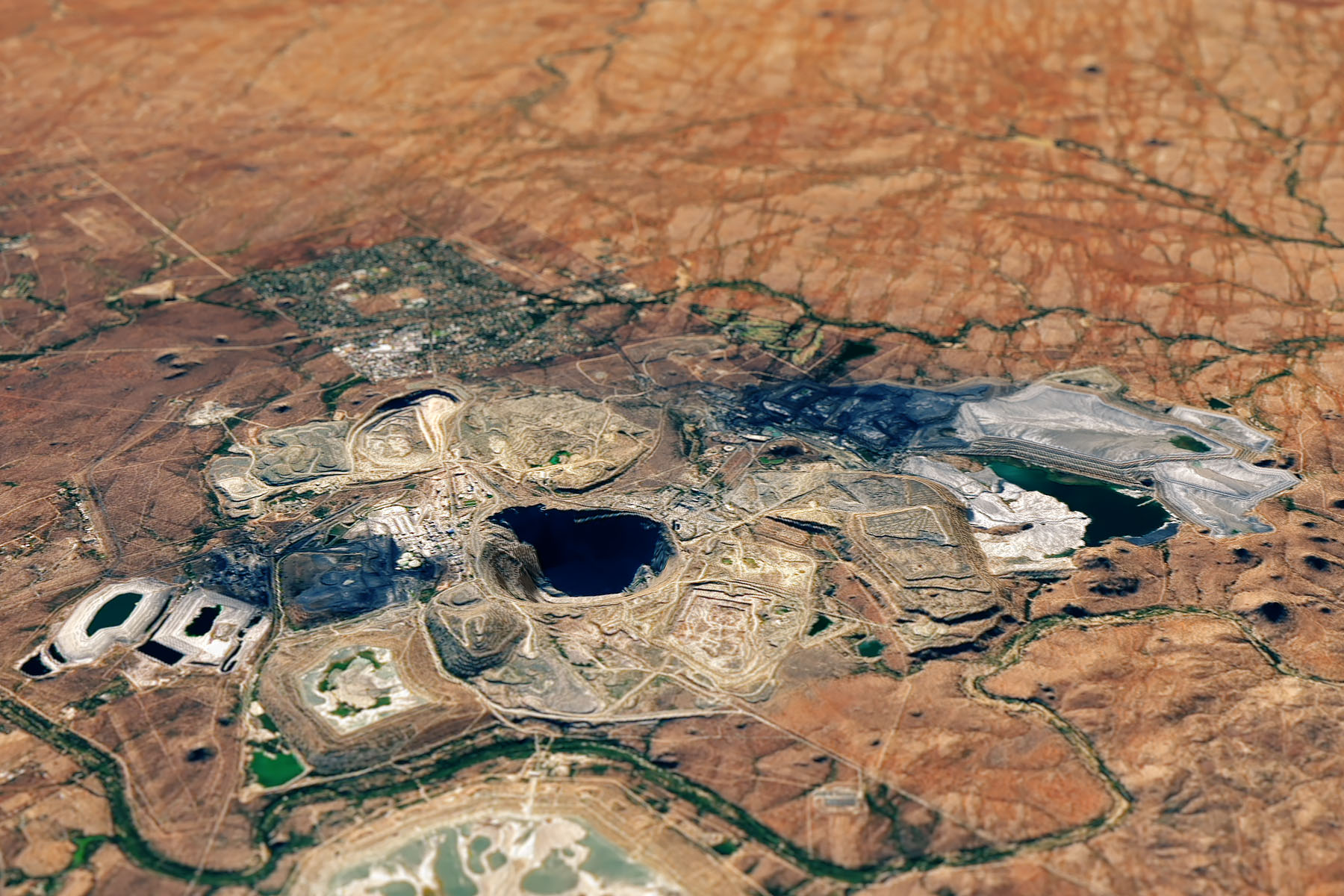This satellite image captures a vast, brown and tan landscape that appears parched, likely due to its arid nature. The area is predominantly bare earth with no visible greenery, hinting at its scarcity of rainfall. The terrain is hilly with various shades of sandy earth, accentuated by a labyrinth of multicolored lines and patches, suggesting a complex industrial site.

At the center of the image is a notable dark circle that might signify a mine or an area heavily excavated and disturbed, surrounded by what seems to be a jumble of interconnected paths and structures. These elements, resembling tangled strings, further imply significant industrial activity.

Scattered throughout the scene, there are patches where a river or creek might have once flowed, now dried up or altered. Within this barren expanse, remnants of small ponds stand out. These water bodies vary in hue—one appears almost green, others are dark blue or have a blackened appearance, likely polluted or affected by industrial processes.

The image suggests a landscape marred by industrial exploitation, with possible sections that have been burned or otherwise destroyed, including areas that might have experienced forest fires. The stark, altered topography is marked by dug-out rock structures and broken spaces, highlighting the extensive human impact on this environment.